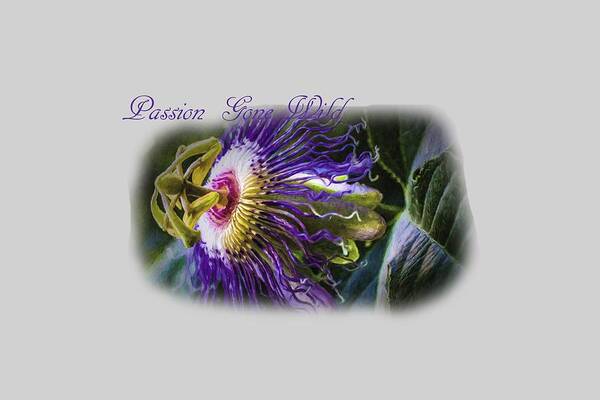In the center of a rectangular image measuring approximately four inches long by three inches tall, there is a digitally created, vibrant flower illustration. The flower, which is somewhat stringy, boasts a striking combination of colors including deep purple, bright pink, pure white, and sunny yellow. The petals extend outward in delicate, noodle-like tendrils, reminiscent of a jellyfish. The center of the flower features a distinct yellow circle, while immediately below it is a vivid pink segment that further transitions into white, blending seamlessly into the surrounding purple petals. The flower appears fully open, with hints of wilting at the petal edges. Adjacent to the flower are large, deep green leaves and a stem with long green arms crisscrossing beneath the bloom. The entire floral display is framed by a wide, plain light gray border. Above the flower, in light purple text, are the words "Passion Gone Wild," adding an expressive touch to the artwork. The overall background is a flat light gray, emphasizing the floral figure at the heart of this creative piece.